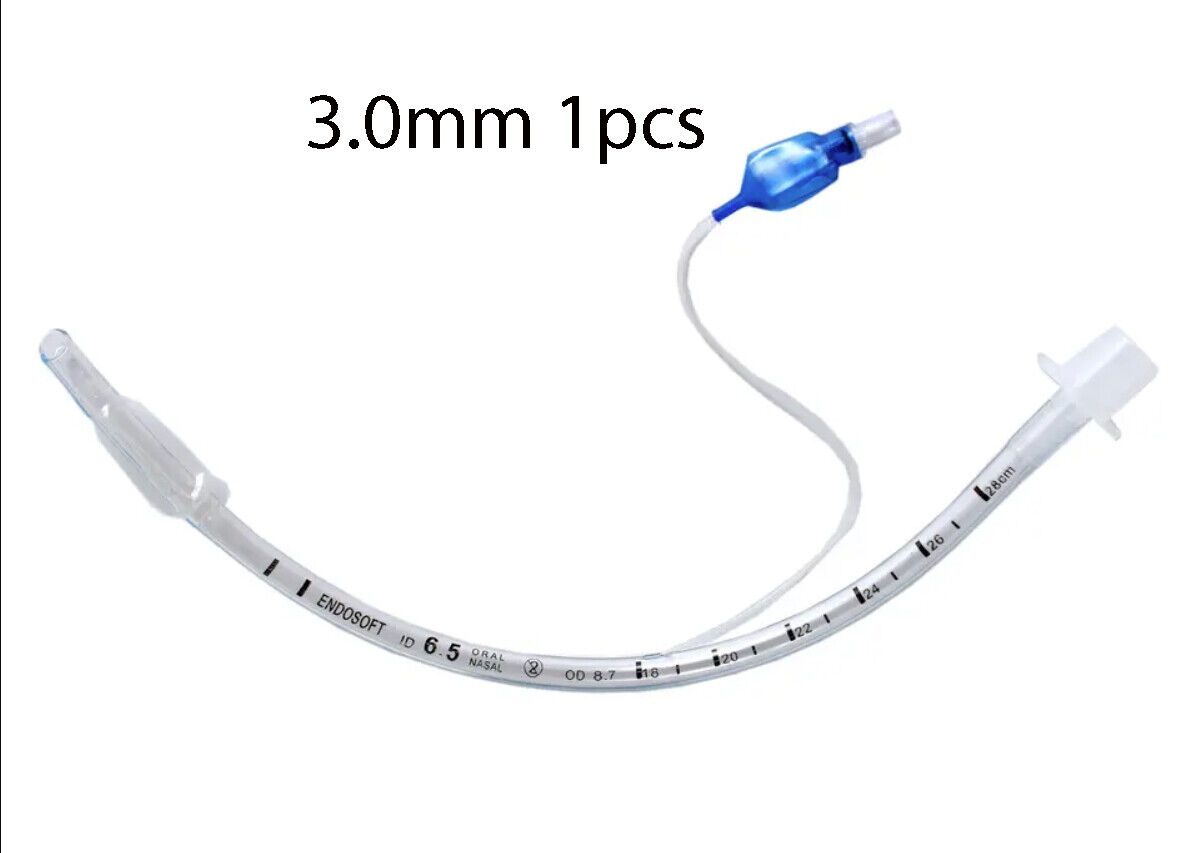The image features a medical apparatus, possibly an Endosoft oral nasal tube, prominently displayed against a white background. The main tube, positioned centrally in the image, forms a U shape with its middle section pointing downwards and curving up both sides. The tube is marked with the text "endosoft 6.5 oral nasal" along with measurements 18, 20, 22, 24, 26, and 28 cm. Above the tube, in black text, it says "3.0mm one pcs." The larger tube is accompanied by a smaller intertwining tube that ascends from the middle, ending with a blue piece that appears to have a fastening mechanism. The apparatus includes a combination of white, black, gray, and blue colors, and features several fasteners. The left side of the image also displays a thin black border line. This medical equipment, likely used in hospital settings for procedures requiring drainage or fluid passage, is meticulously detailed to show its various components and structural design.